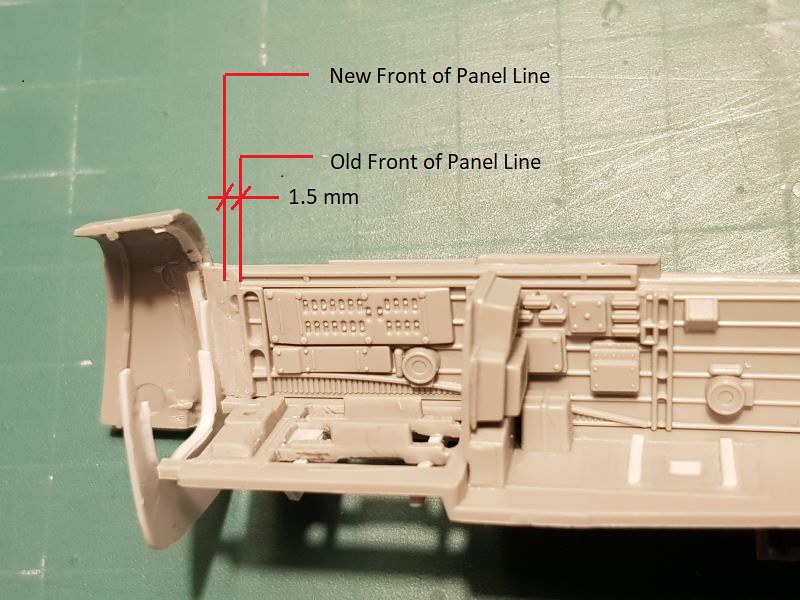The photograph depicts a close-up view of a beige plastic component, possibly die-cast or 3D-printed, resting on a green, grid-lined tabletop. The component features intricate details and annotations in black font, accompanied by three red lines superimposed on the image. The first red line extends from the text "new front of panel line" and connects to the panel. Directly below, another red line extends from the text "old front of panel line" and similarly connects to the panel. A third red line labeled "1.5 mm" intersects the previous two lines, highlighting a 1.5 mm gap between the new and old front panel lines. The overall scene captures the technical intricacies and precise measurements of this plastic device or tool.